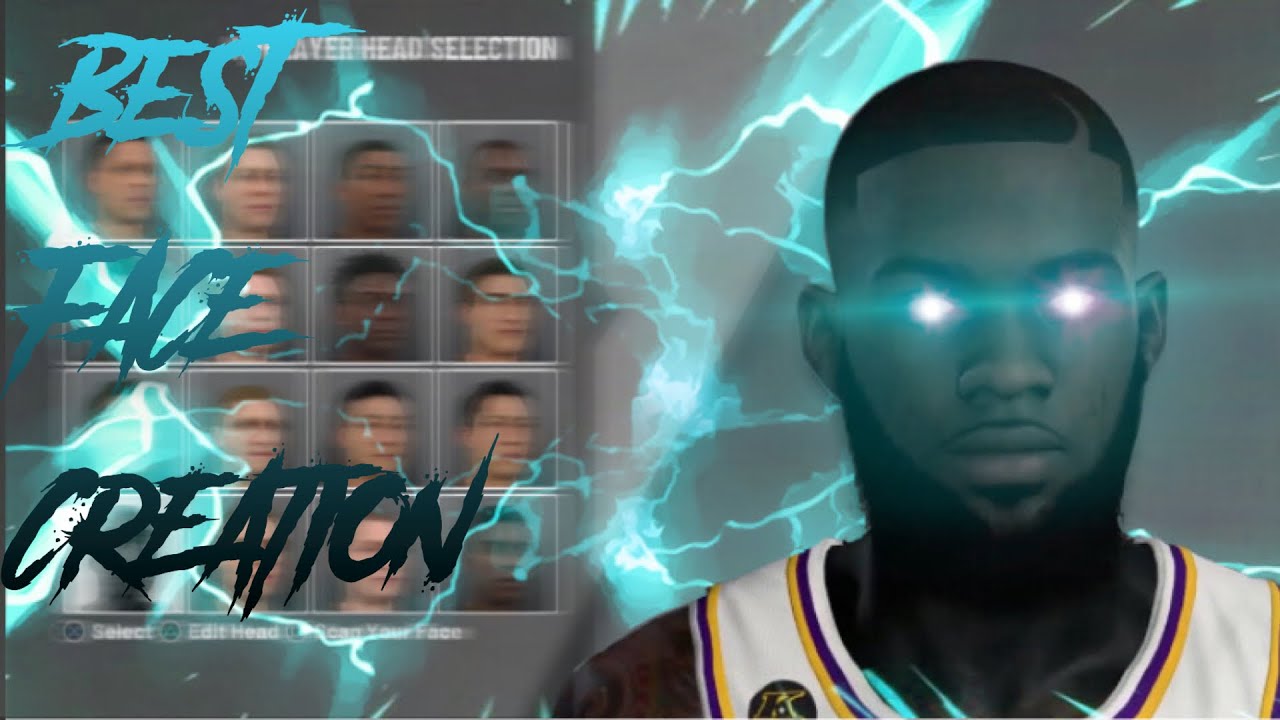This is a highly detailed and immersive character creation interface, likely from a video game. The background is a subdued gray, interspersed with vibrant blue lightning effects that frame the scene from all four sides—left, right, top, and bottom. Dominating the upper portion of the screen, white text labeled "Player Head Selection" is strategically overlapped by a bold, gradient-colored inscription reading "Best Face Creation." This gradient transitions from a light blue to darker blue, culminating in a deep, dark green-blue shade.

The interface showcases a selection grid, arranged in a 4x4 formation, presenting a diverse array of facial options. These faces predominantly represent Caucasian and African American ethnicities, providing a variety of head designs for the player to choose from.

Highlighted on the right side of the screen is a featured character, an African American male with a distinctive appearance. His short hair, beard, slight goatee, and thin mustache are meticulously detailed. This character’s eyes emit a glowing light, adding an enigmatic flair to his overall demeanor. His attire consists of a white jersey adorned with gold and purple trim, indicative of a sporty or futuristic theme. Notably, there is a black circle with a 'K' inscribed within it on the upper right side of his jersey—possibly a logo or insignia. Completing his look, a tattoo is visibly etched onto his right shoulder, adding a final touch of personality and customization.